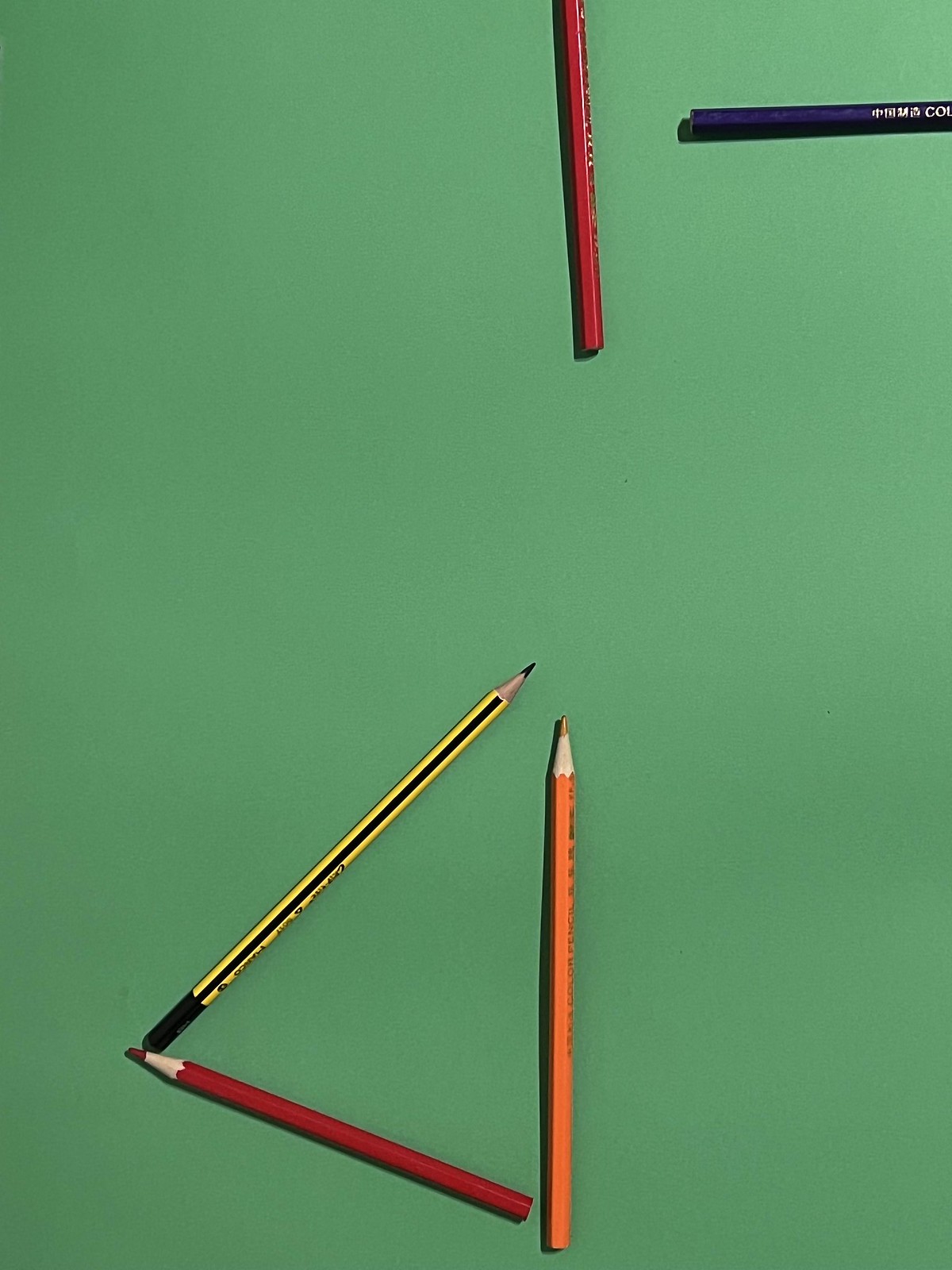The photograph depicts a highly realistic, digitally created image set against a vivid grass-green background. At the top center of the image, a dark red colored pencil is visible, descending from off-frame. To its immediate right, a navy blue colored pencil lies horizontally, marked with indistinct lettering that may include a "C-O-N". The focal point of the image is a triangular arrangement of three pencils towards the bottom portion. This triangular formation, tilted to the right, includes a vertical orange pencil with its tip upwards, a slanted yellow and black pencil to its left with its tip upwards, and a red pencil beneath, pointing leftwards towards the orange pencil. The composition is devoid of people, and the text on the pencils remains largely illegible, contributing to the enigmatic and artistic quality of the scene.